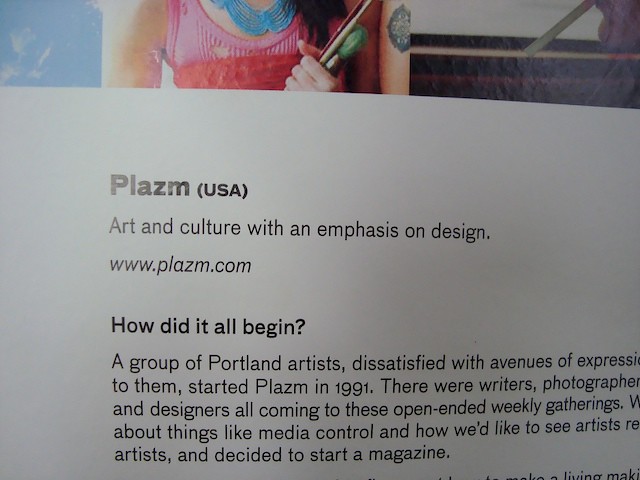The image features a full-color promotional piece. At the top, there is a photograph of a girl partially visible, wearing a sleeveless pink tank top with an orange layer underneath and a bluish necklace. She has a tattoo on one of her biceps and is holding a fistful of paintbrushes. In addition to this photograph, there is an image cut off showing the sky with a few clouds. The background below the images is gray with dark print text that reads, “PLAZM USA Art and Culture with an Emphasis on Design www.plazm.com.” The text narrates how Plazm originated with a group of Portland artists, including writers, photographers, and designers, who, dissatisfied with traditional avenues of expression, began open-ended weekly gatherings in 1991 to discuss media control and envision a new platform for artists. This culmination led them to start a magazine. Some content is cut off, leaving portions of the narrative incomplete.